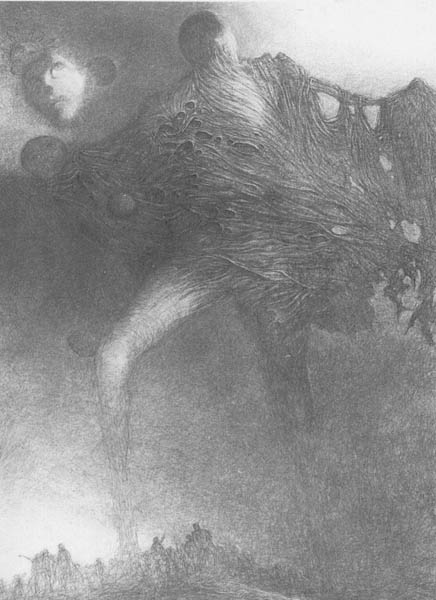This black and white drawing intricately depicts a ghoulish, towering creature with ambiguous facial features, appearing to emerge from a web-like covering resembling yarn or moss. The creature's dark, textured upper torso contrasts with its lighter gray legs, which are positioned as if stepping over a city of small figures and buildings at the base. In the upper left corner, a disembodied head with a face looks on, unconnected to the main figure. The background features circles, reminiscent of planets, adding a cosmic dimension to the scene. This surreal, detailed artwork evokes a sense of an alien or monstrous being, potentially a giant tree-like entity poised to loom over and possibly menace the tiny people below.